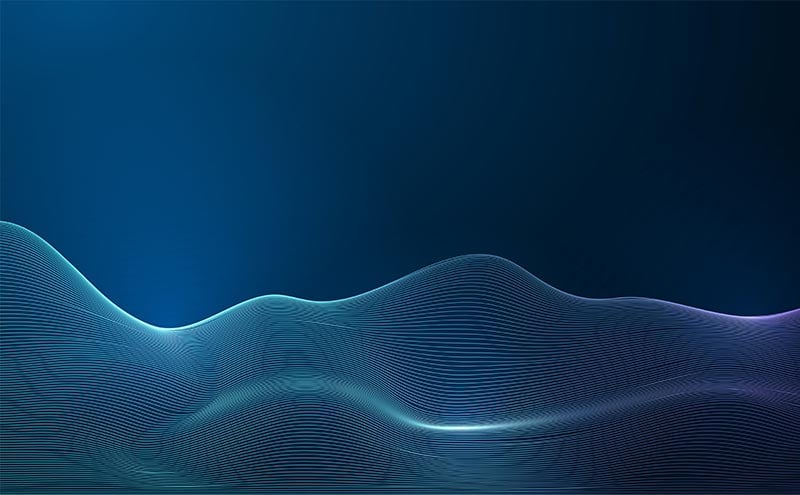The image showcases a striking, abstract design in blue monochrome. The top half features a deep, navy blue background, contrasting with the bottom half, which is dominated by intricate wave-like patterns. These waves are formed by numerous parallel light blue lines, arranged closely together, creating an illusion of swirling patterns within the waves. The interplay of light on these lines adds a luminous quality, with darker blue lines emerging amidst the lighter ones, enhancing the depth and complexity of the design.